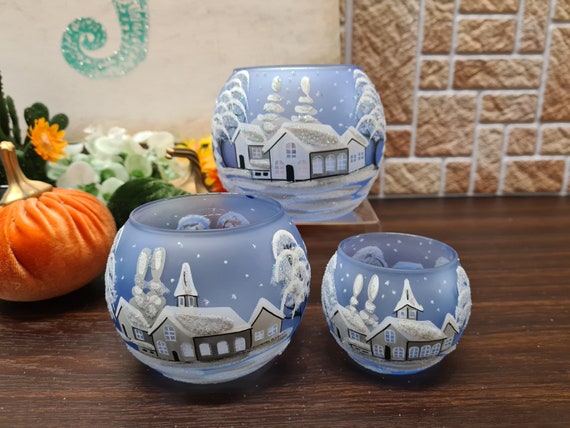The image depicts a close-up of a polished wooden floor composed of two tones of brown, highlighting the natural lines and cracks. Against the wooden floor, there is a two-toned brown and light brown brick wall. Placed on the wooden floor are three round, blue jars, each adorned with detailed winter-themed paintings. The artwork on the jars features a row of snow-covered houses, snowflakes gently falling, tall pine trees cloaked in snow, and a distinct church with additional buildings set against a backdrop of a wintery scene. These jars appear to be candle holders or bowls. To the left of the jars, there's a fabric pumpkin with a golden stem and some decorative flowers. The intricate details on the jars and the juxtaposition of the rustic wooden floor and brick wall create a cozy, wintry ambiance.